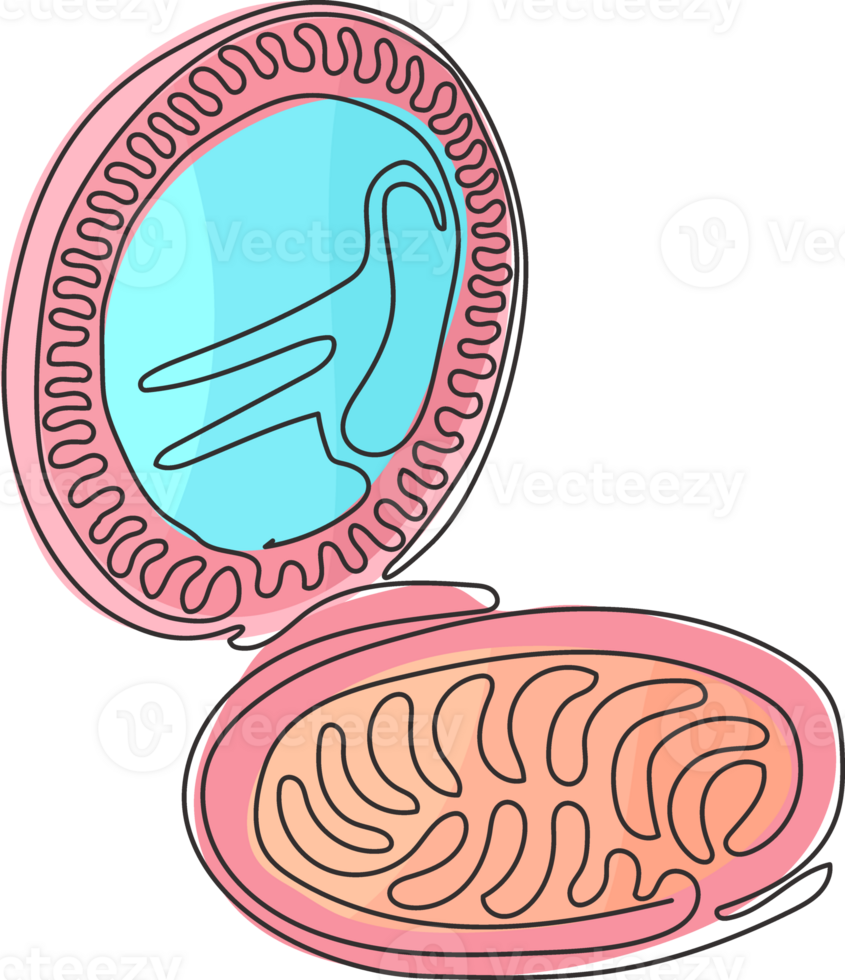This color image resembles a piece of clip art. It features a cartoonish drawing of an open makeup compact, traditionally used by women for holding pressed powder. The body of the compact is painted a cheerful pink, and it has a distinct circular shape. The lower part of the compact, which would typically hold the powder, is colored a salmon orange and is outlined with black ink lines that form an intricate wiggly pattern. The mirror inside the compact is depicted with a light turquoise blue color, surrounded by black outlines and squiggles that create designs resembling a stylized bird with its head down. The paint application is casual, leaving some areas outside the lines, enhancing the playful and artistic feel of the image. A watermark reading "B-E-C-T-E-E-Z-Y" is visible over the art.